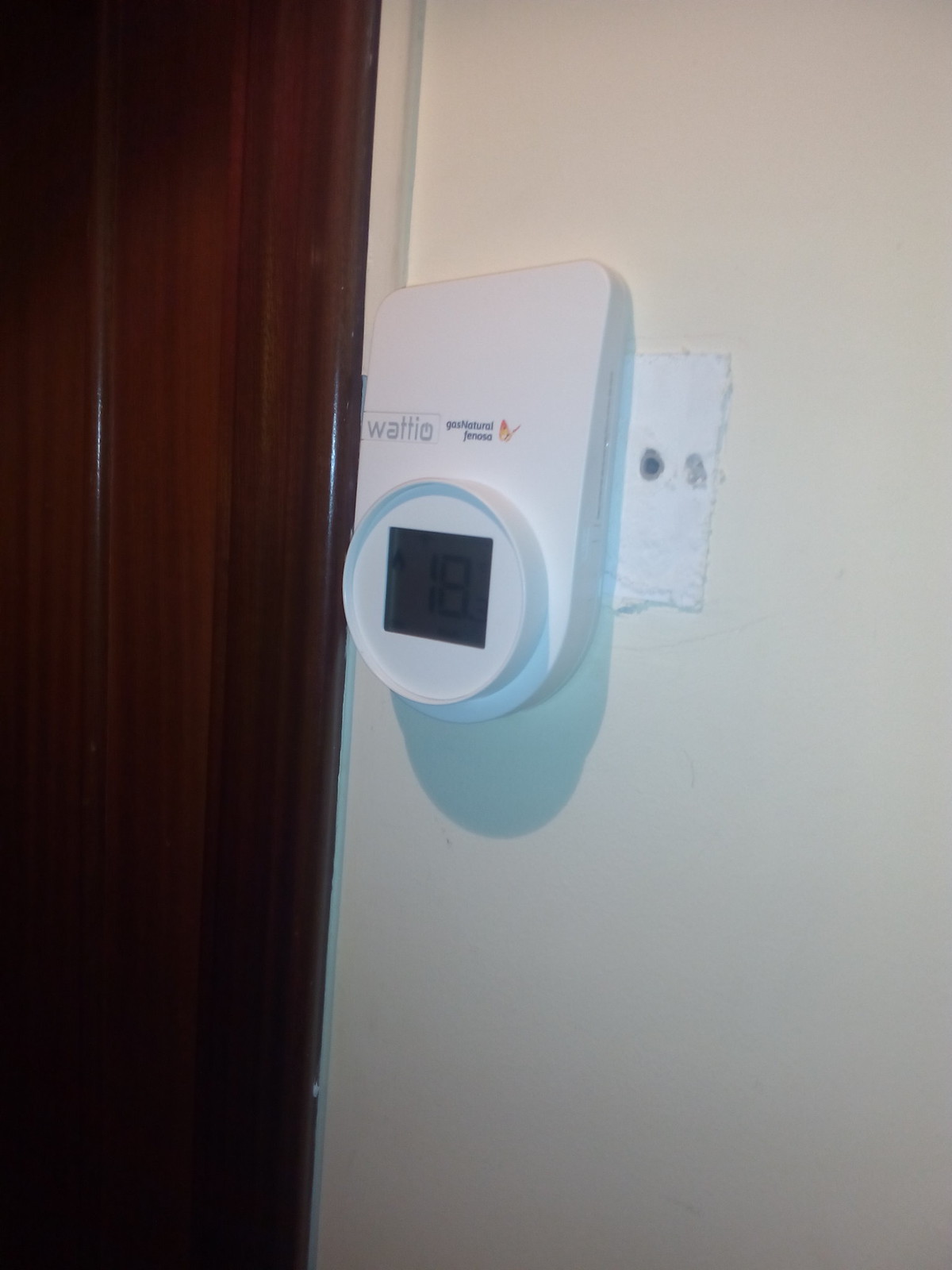The image depicts a close-up view of a digital thermostat mounted on a white wall. The thermostat, which appears to be white in color, prominently displays the brand name "WALI" or "WAITI" in black text. The display screen of the thermostat shows the number "18." The photograph is taken at a slight angle, providing a side view of the device. Adjacent to the thermostat, there is a structure that looks like a door or cabinet, characterized by a brown, wooden finish.